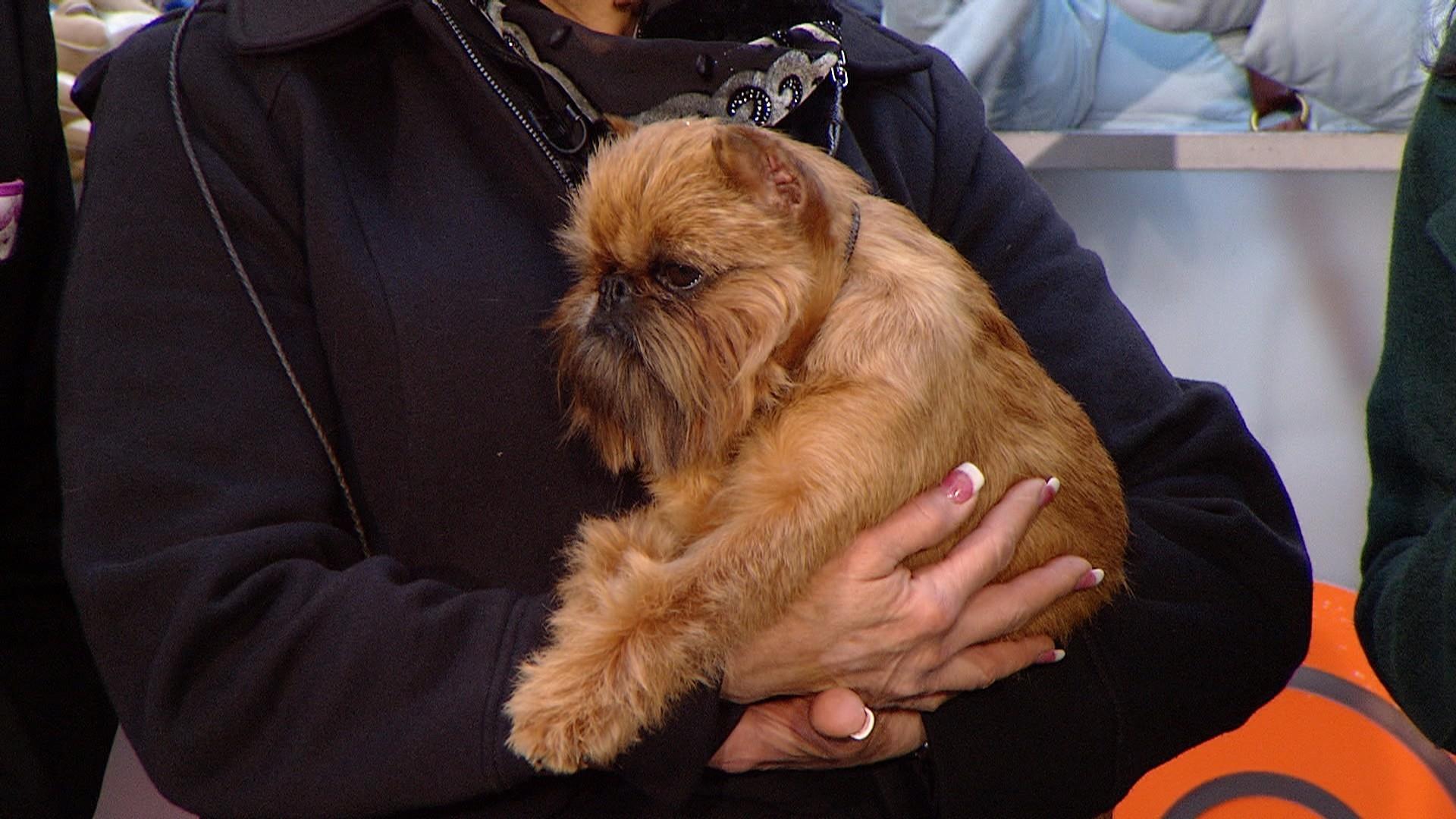In the image, a person is holding a small, brown dog with long hair and a very short snout. The dog has a black nose, dark eyes, and rounded brown ears. The person is dressed in a dark-colored sweatshirt or jacket and is wearing an ornate scarf around their neck. The scarf is black and gray with black crescent moons, adorned with light-colored, shiny stones or sequins. The person has meticulously painted two-tone fingernails, featuring shades of pink and white. They hold the small dog with its paws outstretched, resting comfortably in the crook of their elbow. Behind them, there is a light blue wall that contrasts with other white and light blue objects or materials visible in the background, creating a soft and cozy atmosphere.